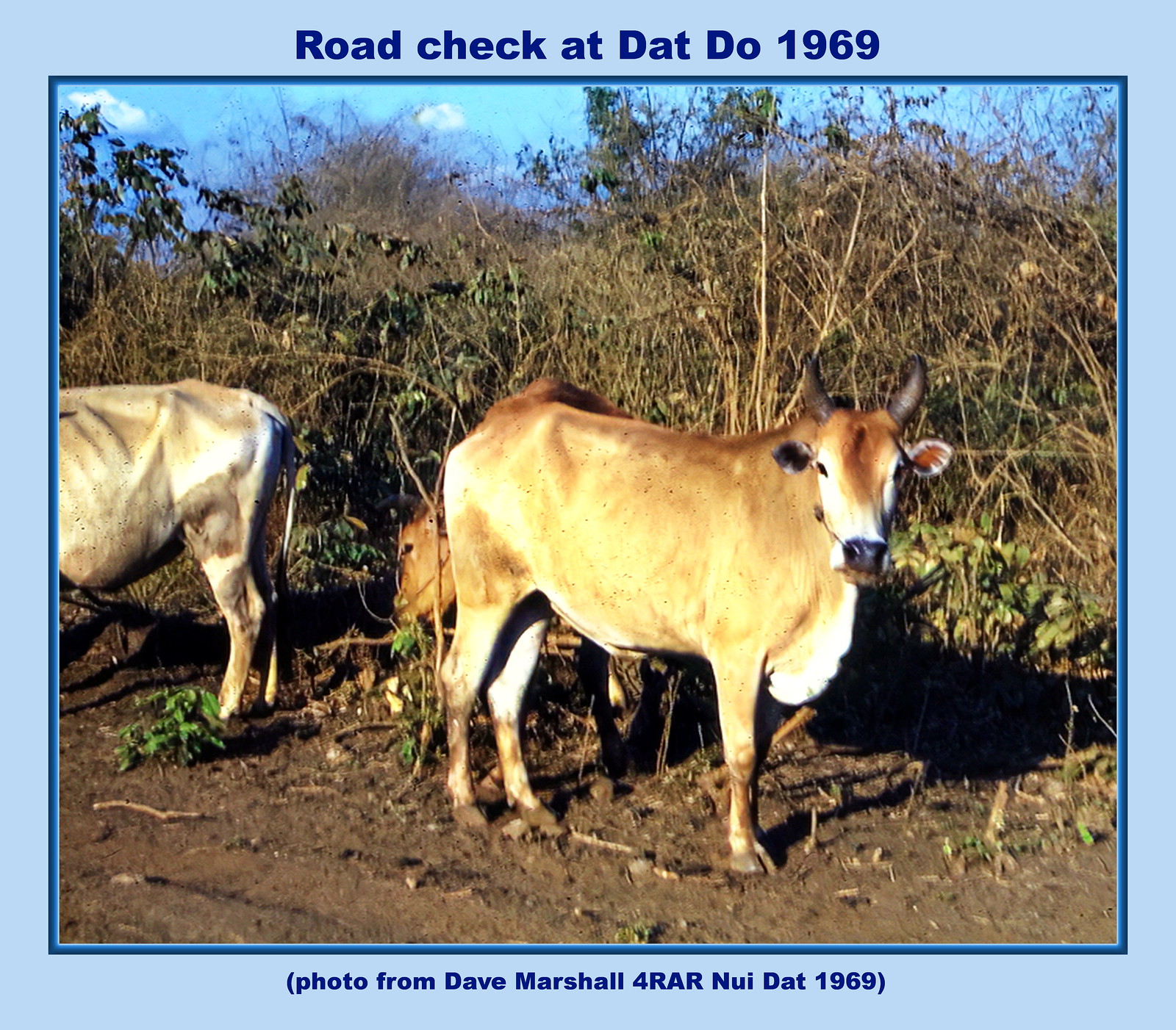This square photo, bordered in light blue with dark blue text, captures a moment labeled "Road Check at Dat Do 1969" on the top, with "Photo from Dave Marshall for RAR Noy Dat 1969" noted at the bottom. The scene features a muddy, brown ground stretching into the background, which is filled with dense, overgrown green plants and brush. In the center of the image, two brown cows stand prominently, with a third cow partially visible on the left side, showing only its abdomen, hind legs, and tail. The sky above is light blue with patches of white clouds, suggesting it’s midday. The cows, possibly bulls due to the medium-length black horns, are either grazing on the bit of grass or standing amidst the muddy terrain. This detailed and vibrant scene captures an outdoor farm-like setting from 1969.